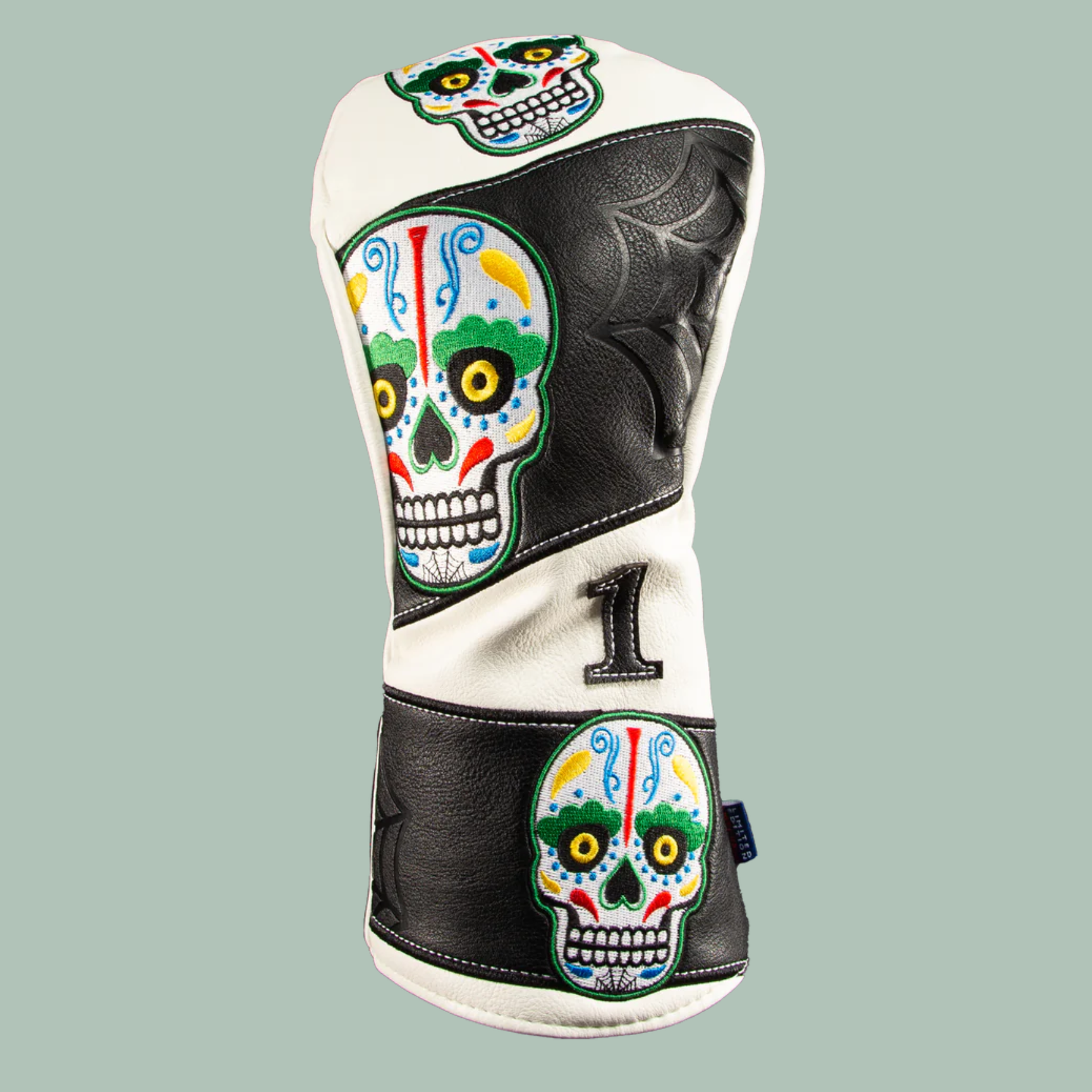The image depicts a leather golf club head cover, intricately designed with a rich array of colors and patterns. Isolated against a moss green backdrop, the primarily white cover features two prominent black stripes, where each stripe is adorned with embossed spider webs. Displayed on the head cover are three ornate, vividly colored skulls that resemble Mexican Day of the Dead motifs. Positioned at the top, middle, and bottom, the middle skull is noticeably larger than the other two. Each skull is meticulously detailed with yellow eyes encircled by green, a distinctive red line—styled like a golf tee—running down the forehead, flanked by blue and yellow squiggly lines, and complemented with a white-toothed grin, red, blue, and yellow accents around the mouth, and a subtle spiderweb design on the chin. A black number "1" with white stitching is also prominently featured. The entire protective cover exhibits a unique blend of artistry and functionality.